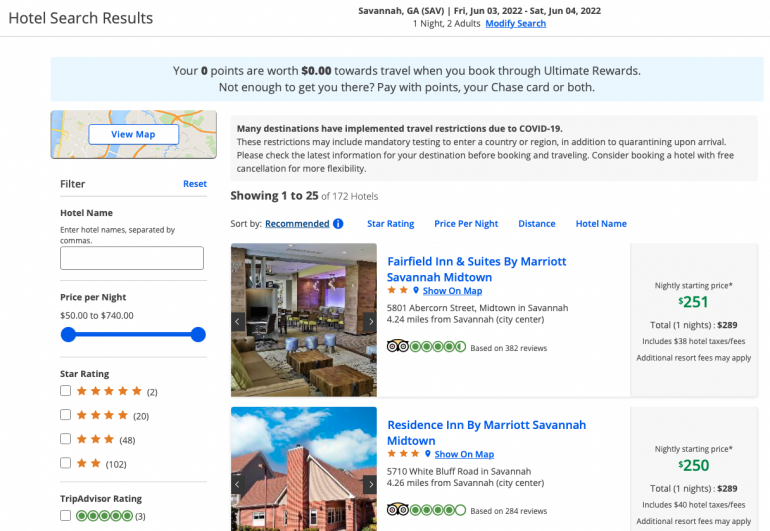This is a detailed screenshot from Google, showcasing hotel search results for Savannah, Georgia. The search parameters are displayed prominently, indicating a booking for one night from Friday, June 3, 2022, to Saturday, June 4, 2022, for two adults. A blue banner at the top mentions, "Your 0 points are worth $0 towards travel when you book through Ultimate Rewards." In the top left corner, there's a "View Map" section, followed by various filtering options that allow users to sort by hotel name, price per night, star rating, and TripAdvisor rating.

Below the filtering options, the main content starts with a gray banner alerting users about potential COVID-19 travel restrictions. The page is displaying hotel results 1 to 25, sorted by recommended options.

### Featured Hotels:
1. **Starfield Inn and Suites by Marriott Savannah Midtown**
   - **Rating:** 2 stars
   - **TripAdvisor Rating:** 4.5/5 based on 382 reviews
   - **Price:** $251 per night, including hotel tax fees
   - **Image:** The inside lobby
   - **Other Details:** The hotel's address and its distance from Savannah are noted.

2. **Residence Inn by Marriott Savannah Midtown**
   - **Rating:** 3 stars
   - **TripAdvisor Rating:** 4/5 based on 284 reviews
   - **Price:** Starting at $250 per night
   - **Image:** The exterior of the property
   - **Other Details:** A "Show on Map" link is available, along with the hotel's address and its distance from Savannah.

This comprehensive view provides travelers with essential information to make an informed hotel booking decision.